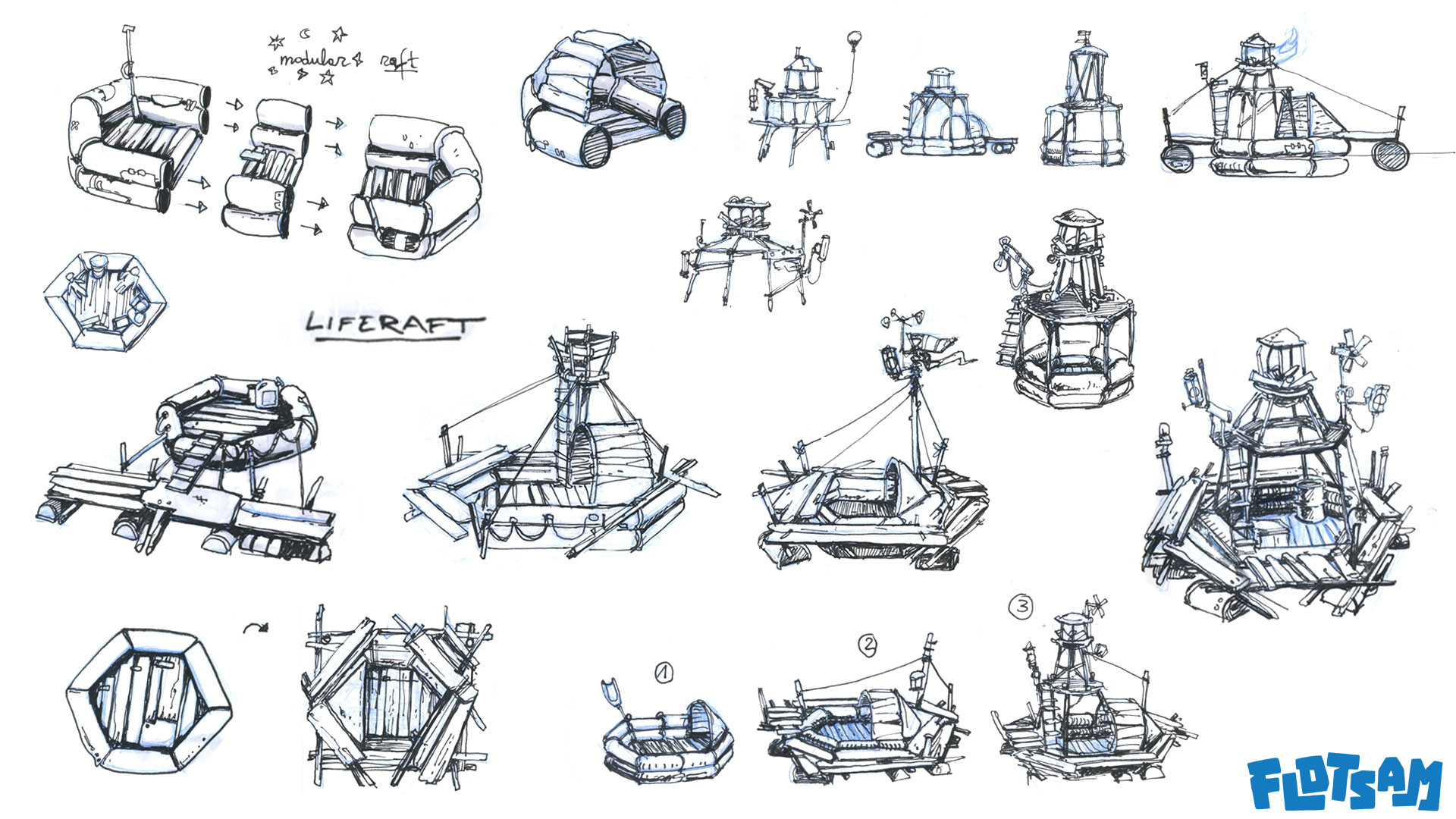This image showcases an intricate drawing depicting the construction and evolution of various floating vessels, progressing from simple rafts to more complex boats and ships. The artwork is composed of approximately 20 smaller drawings, each illustrating a different stage of assembly. The detailed illustrations vary, with some showing fully built boats while others depict early construction phases. The left side prominently features a life raft, and the bottom right corner includes the word "Flotsam" in stylized, cartoonish blue lettering. While the majority of the drawings are rendered in black and white, select elements, such as water and certain boat parts, are highlighted in shades of blue, adding depth and contrast to the piece. This meticulously detailed artwork beautifully captures the essence of maritime construction.